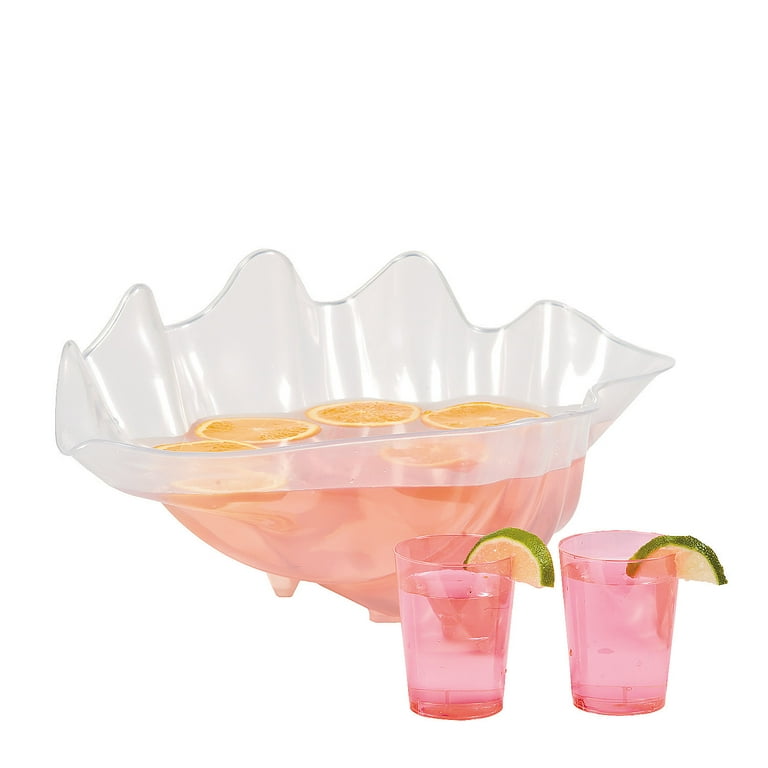The image features a striking punch bowl crafted in the shape of a sea scallop, exuding elegance with its scalloped top edge and typically translucent or pearlescent finish. The large punch bowl, which can hold over 20 servings, is filled with a light pink liquid. Floating atop the drink are five slices of orange, adding a touch of vibrant color. In front of this majestic bowl are two matching pink glasses—either acrylic or glass—each approximately 5-6 full of the same pink drink, complete with a lime slice garnish on the rim. The entire scene is set against a completely white background, emphasizing the freshness and inviting look of the punch.